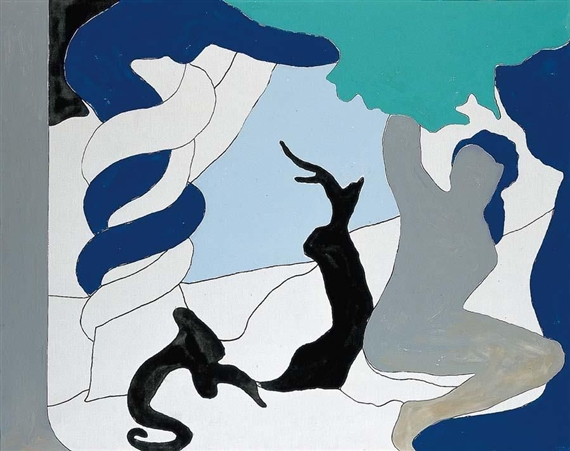This abstract painting visually interprets the Garden of Eden with a minimalistic and stylized approach. Dominated by muted and cool tones of gray, blue, green, and white, the left side of the composition features a thick vertical bar of gray. To the right, a simplified yet recognizable silhouette of a woman, depicted in gray with blue hair, stands reaching towards a tree. This tree, central in the artwork, has teal-colored leaves and black roots, with a blue and white snake coiled around its trunk, symbolizing the biblical serpent. Though minimalistic, the use of color and form effectively conveys the scene's essence, with the abstracted woman appearing naked, her figure blending into the ambiguous white background, which may also suggest the presence of stones or grass on the ground. The overall piece balances detail with abstraction, utilizing stark contrasts and subtle hues to represent the iconic biblical tale, Eden.